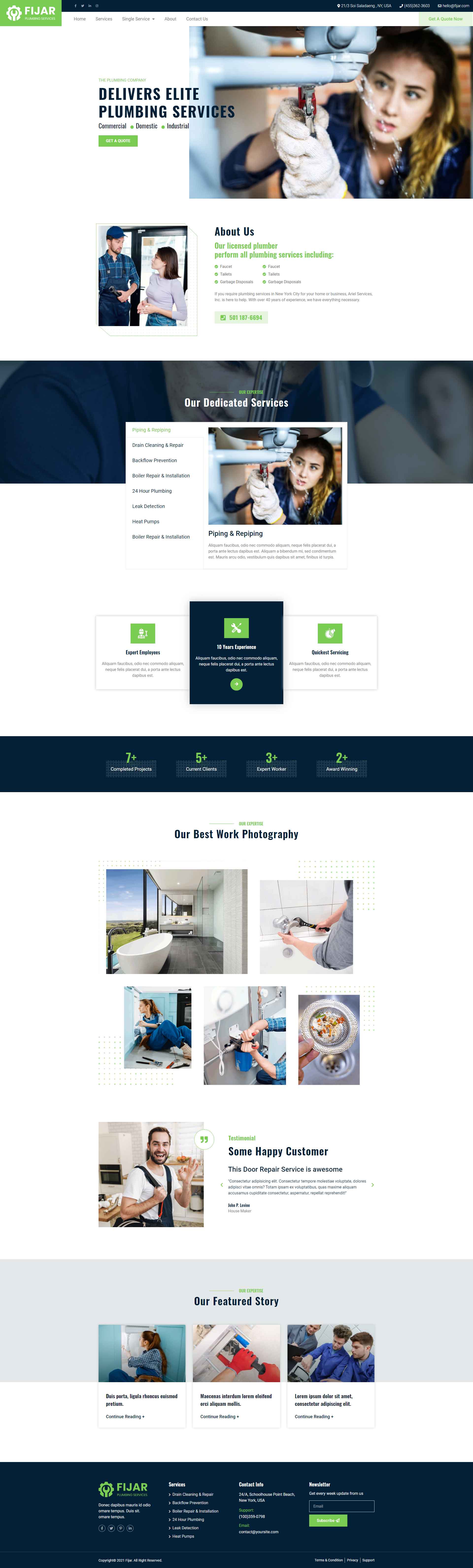The image appears to be a screen capture from a website. At the top, there's a black header bar featuring a green rectangle in the upper left-hand corner, which likely serves as the website's logo or a navigation element. Below it, the main background is white.

In the upper right corner, there's a large image of a female figure with brown hair, wearing white gloves, and working on a pipe. To the left of this image is some text that reads, "Delivers Elite Plumbing Services," with a green call-to-action button positioned right below the text.

Underneath, there is a smaller picture showcasing both a male and a female, with accompanying text on the right side. Continuing downward, there is a gray-bordered section, faintly visible due to a white pop-up overlay, which features the same image of the female working on the pipe.

Beneath the pop-up, three square elements are visible: two white squares sandwiching a black square in the center. Each square contains a green rectangular button.

Further down, there's another black border followed by a white section featuring five grouped images with text below them and a smaller image to the left of this text. 

Finally, the bottom part of the screen comprises a gray area containing three small rectangular pictures, and at the very bottom, a black section loaded with text, which seems to be information on how to contact the business.